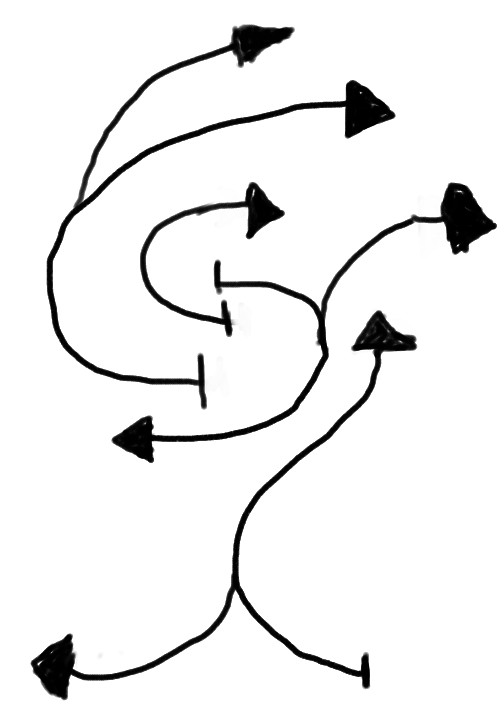This image features a drawing on an all-white background, likely created using a black marker on a dry erase board, as suggested by the visible smear lines on some of the strokes. The artwork is a complex collection of lines with various terminal shapes. 

Starting from the bottom, there is a single line that splits into a Y shape. The left branch of the Y ends in a sharp, pointed triangle, while the bottom right branch remains as a simple line.

Moving upwards to the central area of the composition, another line also splits into a Y shape. This branch has a pointed triangle at the bottom and a rounded triangle shape on the top right, with a straight line forming the top end.

Towards the top center, a different single line features a spear-shaped tip on one end and a block-like horizontal line on the other. 

Another singular line in the image has a vertical line on one end, which then splits into two at the top. One end of this split finishes with a thin, spear-like tip, while the other terminates in a broad, large triangle.

Overall, the drawing showcases a variety of geometric forms and intricate intersections, all rendered in stark black on the white canvas of the dry erase board.